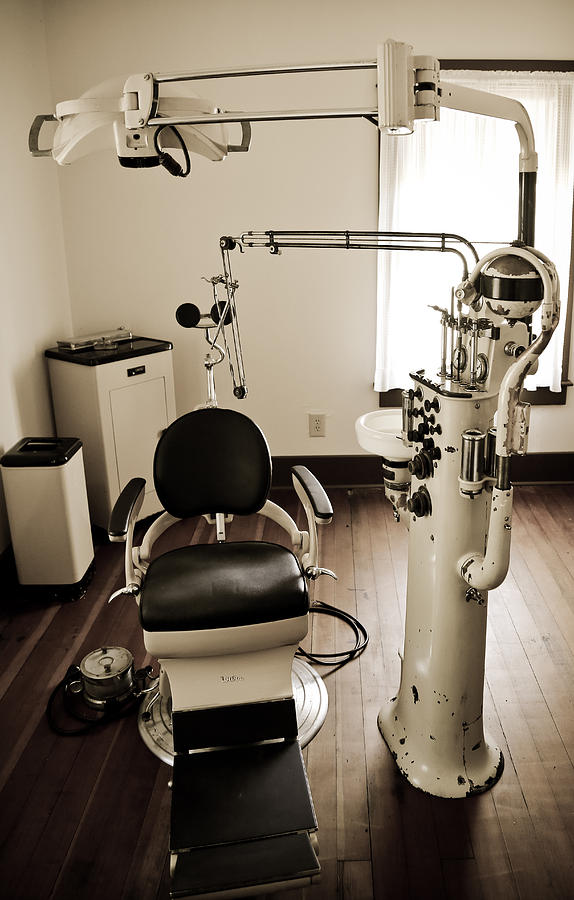This image depicts a detailed scene inside what appears to be a medical office, possibly belonging to an optometrist or a dentist. Dominating the center of the room is a white chair with black leather upholstery in areas where the body contacts the seat, designed to recline and adjust in height. To the immediate right of the chair stands a sophisticated white and black machine that features various attached devices and what seems to be a small sink, indicating its use for patient examinations.

The room's background showcases two matching white tables topped with black surfaces, positioned along beige walls and a large white-curtained window through which sunlight streams, casting reflections on the dark brown hardwood floor. There is also a singular electrical outlet visible on the gray-toned wall. The meticulous arrangement and color scheme of white and black, along with functional medical equipment and furnishings, provide a clean, professional atmosphere suitable for a healthcare setting.